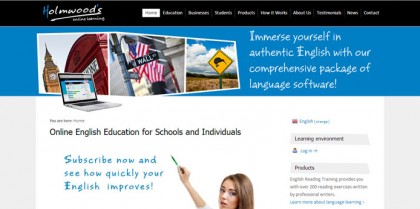The image depicts a screenshot of a website named HolmWoods. The website's name, "HolmWoods," is prominently located in the top left corner of a black header. Alongside HolmWoods in the header, there is a menu bar, though the text in the menu is too small to be clearly legible. The upper section of the webpage features a blue background, transitioning to a gray background below.

Within the blue section, there are three Polaroid-style images arranged side by side. The central image showcases Wall Street adorned with American flags. To the left, there is a picture of London with Big Ben and a traditional red telephone booth. The right image depicts a street sign featuring what appears to be a kiwi, suggesting a New Zealand bird.

To the right of these Polaroid images, a text reads, "Immerse yourself in authentic English with our comprehensive package of language software." Adjacent to this, in the white section of the webpage, the title "Online English Education for Schools and Individuals" is displayed. Below this title, blue text encourages users to "Subscribe now and see how quickly your English improves."

Additionally, there is an image of a female teacher writing on a wall, reinforcing the educational theme of the website. On the right side of the page, tabs for "Products" and "Learning Environment" are present, providing further navigation options.